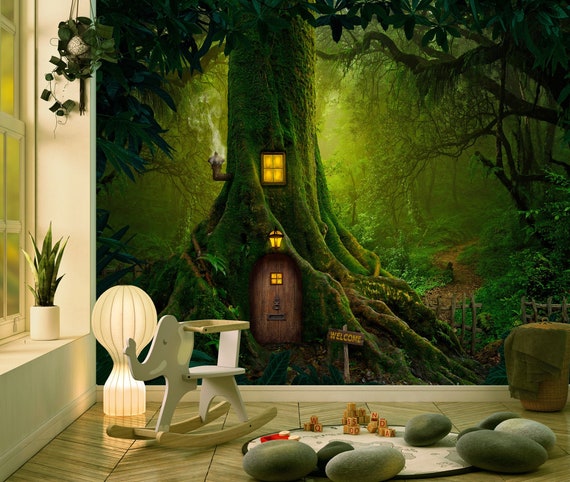The image portrays a cozy nursery room featuring a tan floor with V-shaped or zigzag designs. Prominently, there is an enchanting wallpaper that depicts a lush green tree with vibrant foliage. At the base of the tree, there is a tiny, warmly lit door that seems to invite a little elf, accompanied by a welcoming sign and a quaint chimney peeking out above the tree trunk. The scene inside the nursery includes a gray elephant-shaped rocking chair positioned to the left and a white circular carpet adorned with gray, rock-shaped pillows. A window on the left side of the room allows natural light to softly illuminate the space, creating a whimsical and inviting ambiance.